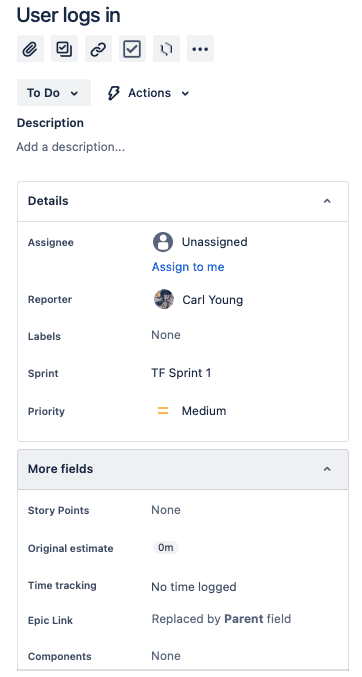Screenshot Description:

This screenshot appears to be taken from a mobile phone, suggested by its long, vertical format. The interface displays a user-centric program, predominantly featuring a white background with black text, accented by elements of blue and a small orange icon.

At the top, the header reads "User Logs In." Following this, there's a row of various icons, including a paper clip, a check mark, a chain link icon, another check mark housed within a box, a pair of brackets, and three vertical dots, indicating additional options.

Below these icons is a section with the label "To Do," followed by "Actions." The section titled "Description" prompts users to "Add a description." This is followed by the "Details" section, which appears to be expanded.

In the "Details" section:
- **Assignee:** Unassigned, with an option in blue text to "Assign to me."
- **Reporter:** Carl Young, alongside a small avatar photo.
- **Labels:** None.
- **Sprint:** TF Sprint 1.
- **Priority:** Marked as Medium, indicated by the small orange icon.

Further details include a "More Fields" section showing:
- **Story Points:** None.
- **Original Estimates:** 0 hours.

At the bottom of the screenshot, a link to "More info" is provided for additional details.